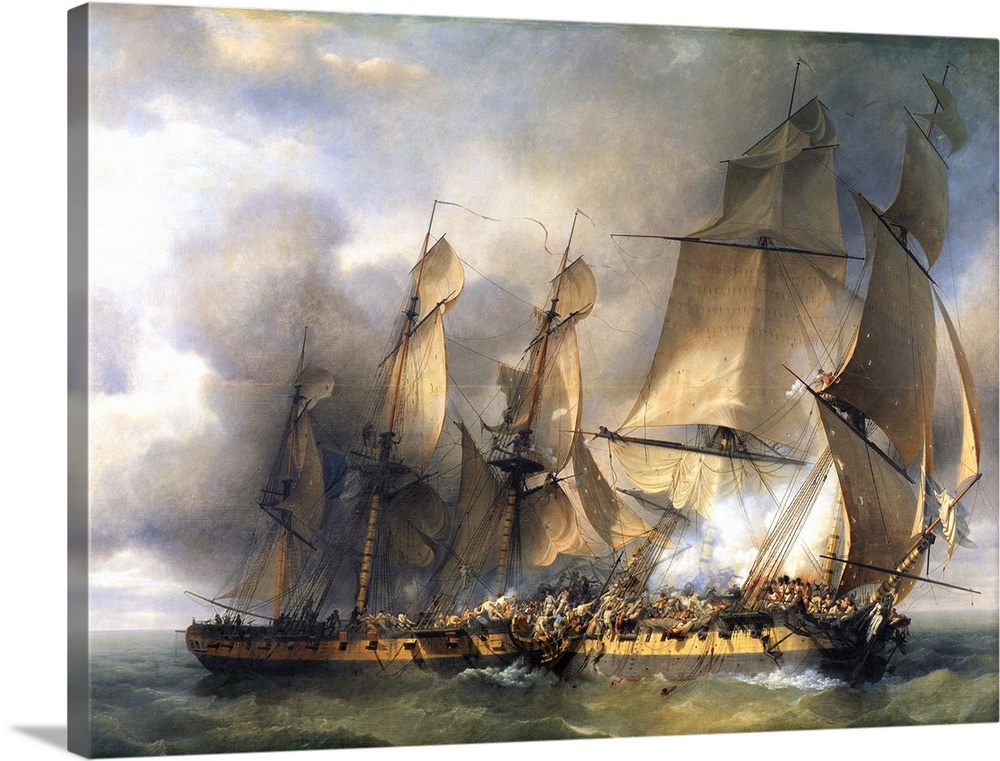This detailed oil painting, likely a canvas print as noted by its visible 3D edge and shadow, depicts a dramatic maritime scene. At the center of the composition are two masted ships, both with intricate sails and rigging. The left ship boasts five masts adorned with complete sails, while the right one, seemingly in distress, has only two masts. These vessels share similar color schemes, featuring black bottoms and yellow trim along the deck where rows of cannons are visible. 

The scene is enveloped in a stormy atmosphere, with dark, tumultuous clouds dominating the sky and only occasional patches of blue breaking through. The sea below them is choppy and active, adding to the tension. Smoke rises from the right ship, suggesting an ongoing calamity—either an attack or perhaps a rescue attempt.

Both ships are teeming with people, creating an impression of chaos. Some individuals are seen overboard, emphasizing the perilous situation. The sails on both ships are in disarray, flapping wildly in the wind, further contributing to the sense of urgency and struggle. The close proximity of the ships intensifies the scene's dramatic effect, leaving the viewer to ponder whether they are adversaries or allies in a desperate scenario at sea.